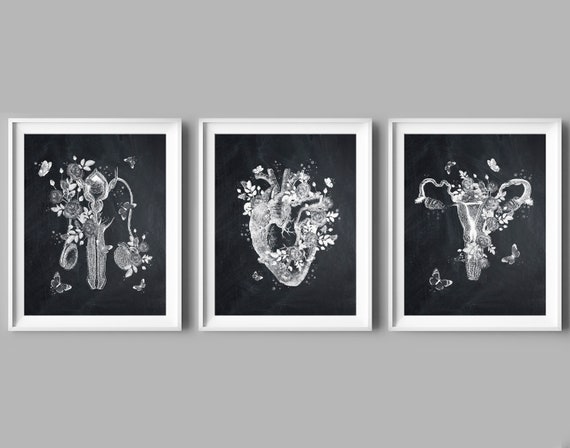The image depicts three framed illustrations hanging on a gray wall. Each frame is white with white matting, and the illustrations inside have black backgrounds with detailed white and gray artwork. The first illustration appears to be an abstract representation of the male reproductive system, adorned with flowers, leaves, and butterflies. The middle illustration, an abstract depiction of a human heart, is similarly embellished with flowers and butterflies. The third illustration portrays the female reproductive system, featuring fallopian tubes and ovaries, also surrounded by butterflies and flowers. Each piece shares the same artistic style, combining anatomical elements with intricate floral and butterfly motifs.